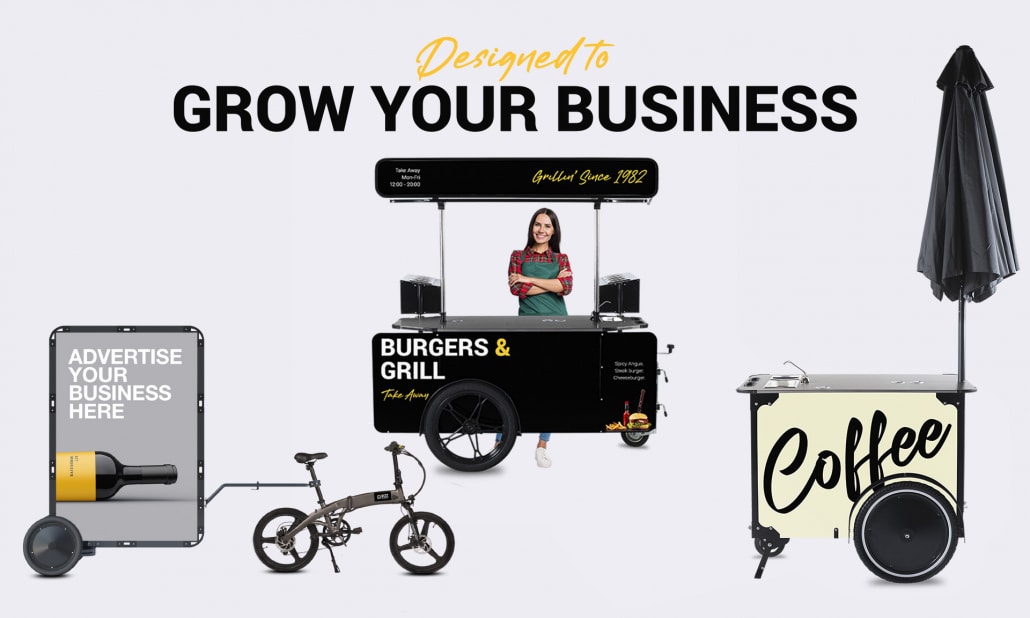The image depicts an advertisement titled "DESIGNED TO GROW YOUR BUSINESS" with "Designed to" in small green letters and "GROW YOUR BUSINESS" in large black, all-capital letters. Centered in the image is a black burger and grill cart labeled "BURGER AND GRILL" in white and yellow lettering, with the tagline "GRILLING SINCE 1982" written in white on its black top. Behind the cart stands a smiling Caucasian woman wearing a green apron over a red plaid shirt, with her arms folded. To the right of the cart is a portable coffee stand with an umbrella, and to the left, there is a child's bicycle pulling a marquee on wheels that reads "ADVERTISE YOUR BUSINESS HERE" in white letters. The backdrop is a light blue color, and the overall impression is that the image serves as an advertisement for a service that offers promotional space on mobile food carts and portable billboards.